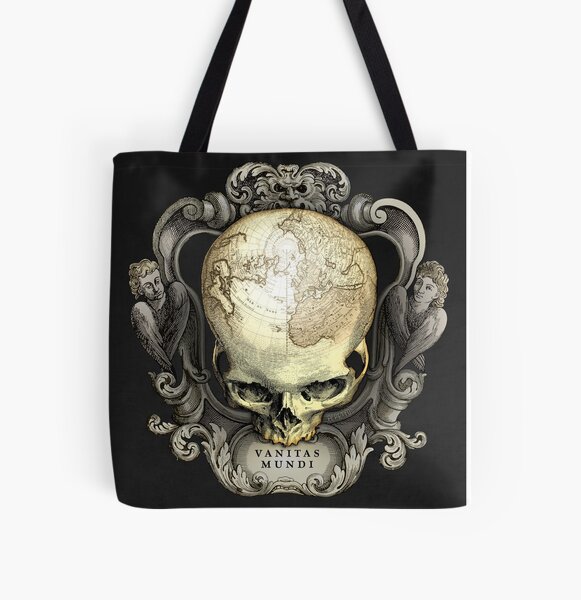This color photograph captures a black women's tote bag hanging against a light gray background. The tote bag, partially cut off at the top where the straps extend beyond the frame, features a detailed illustration in the center. The artwork shows a skull viewed from above, its surface adorned with an Old World map. The skull, rendered in a light off-white color reminiscent of aged stone, also has identifiable eye and nose sockets. Surrounding the skull is ornate scrollwork, which frames two cherubs or angels, each positioned opposite the other with faces turned outward and wings crossed in front. At the bottom of the bag, the text "Vanitas Mundi" is prominently displayed.